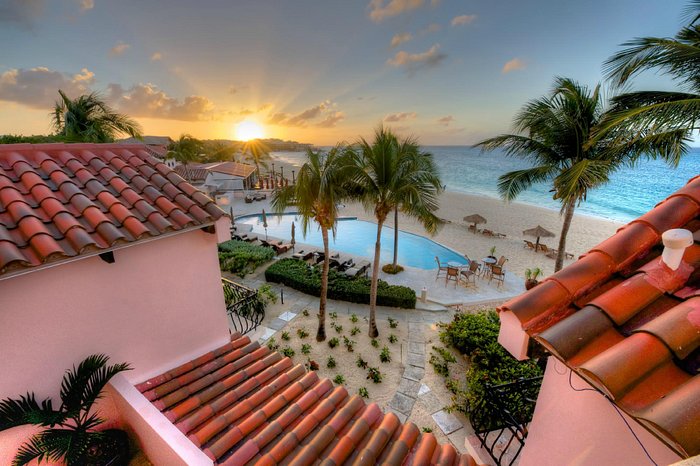This detailed photograph captures a serene sunset at a beachside resort, viewed from a rooftop cabana area. Dominating the foreground are three shingled rooftops, their curved surfaces featuring red and pink hues. The walls below are painted a matching pink. To the left, a tall palm tree stretches upwards while numerous other palms are scattered around the scene, their leaves rustling in what appears to be a gentle breeze. Below, a sandy beach transitions into a large, oval swimming pool encircled by a gray cement deck. Nearby, lounge chairs and bar stools with tables invite relaxation, though there are no people present. The tranquil ocean lies to the right, its blue waters blending into the horizon. Off in the distance, the setting sun emits rays of orange and yellow light, casting a warm glow across the sky and the few scattered clouds. The picturesque resort ambiance is further enhanced by the presence of more distant buildings, black railings, a meandering sidewalk, and well-maintained gardens.